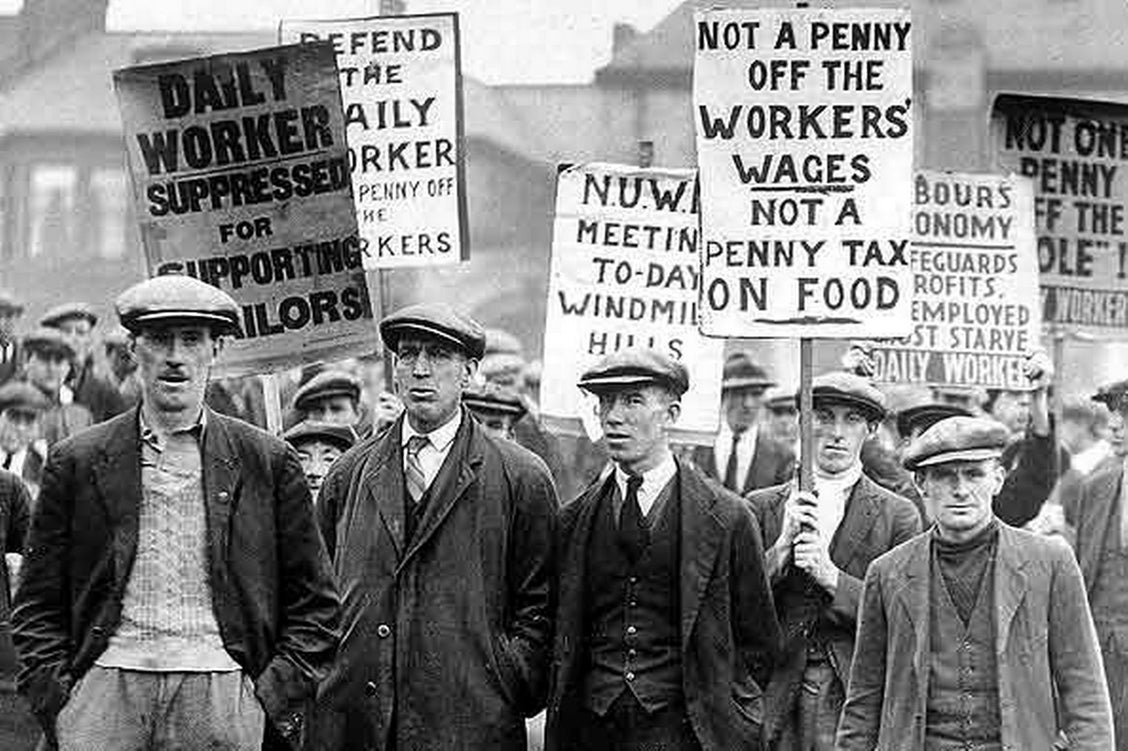This black-and-white photograph, likely taken during the Great Depression or early 1900s, depicts a large crowd of men engaged in a union labor strike. The men, dressed in suits and round black hats, are holding various protest signs with slogans like "Not a penny off the workers' wages," "Not a penny tax on food," "Daily worker suppressed for supporting sailors," and "NUW meeting today." The scene is bustling with dozens of men, all focused on their cause. In the background, houses and possibly factory buildings are visible, adding context to the workers' struggle. The sky appears white, indicative of daytime and the limitations of black-and-white film. The photograph shows signs of compression artifacts, highlighting its age and the technology of the time.